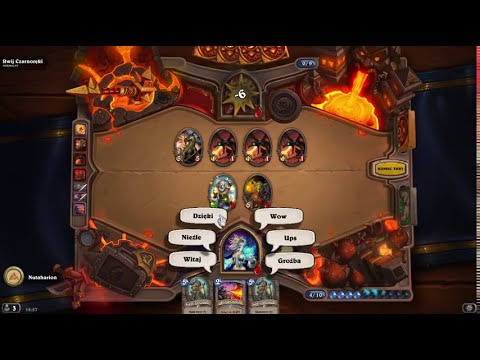The screenshot captures a detailed view of a video game that resembles a card or strategy game. The image features a horizontal black border at both the top and bottom, framing the scene. The central play area is depicted as a tan-colored surface, reminiscent of a game board or table. 

In the corners of this board, various thematic elements are present:
- The top left corner shows rocks amid flowing lava, with a gold spear piercing through them.
- The upper right corner depicts a monstrous stone figure spewing lava into a pool below.
- The bottom right corner contains indistinct dark objects, possibly crates or cases.
- The bottom left corner houses a black chest.

Dominating the center of the screen are four oval icons, likely representing characters or important game elements, arranged in a row across the middle. Below this set of four, two more circles can be seen, creating a secondary row. Between the top corners, an olive-colored starburst displays a "-6," possibly indicating some sort of counter or score. 

Further down, below the oval icons, a shield-shaped area is present with word bubbles exclaiming phrases like "WOW," "UPS," and "WICKEDGE," emanating from an arched window. 

At the very bottom, three cards reminiscent of Yu-Gi-Oh or Pokémon cards, each adorned with distinct characters, lie in a horizontal row. The layout suggests a competitive match, potentially between two players. The entire scene is set against a blue background with gold stripes on either side, adding to the overall immersive and dynamic atmosphere of the game.